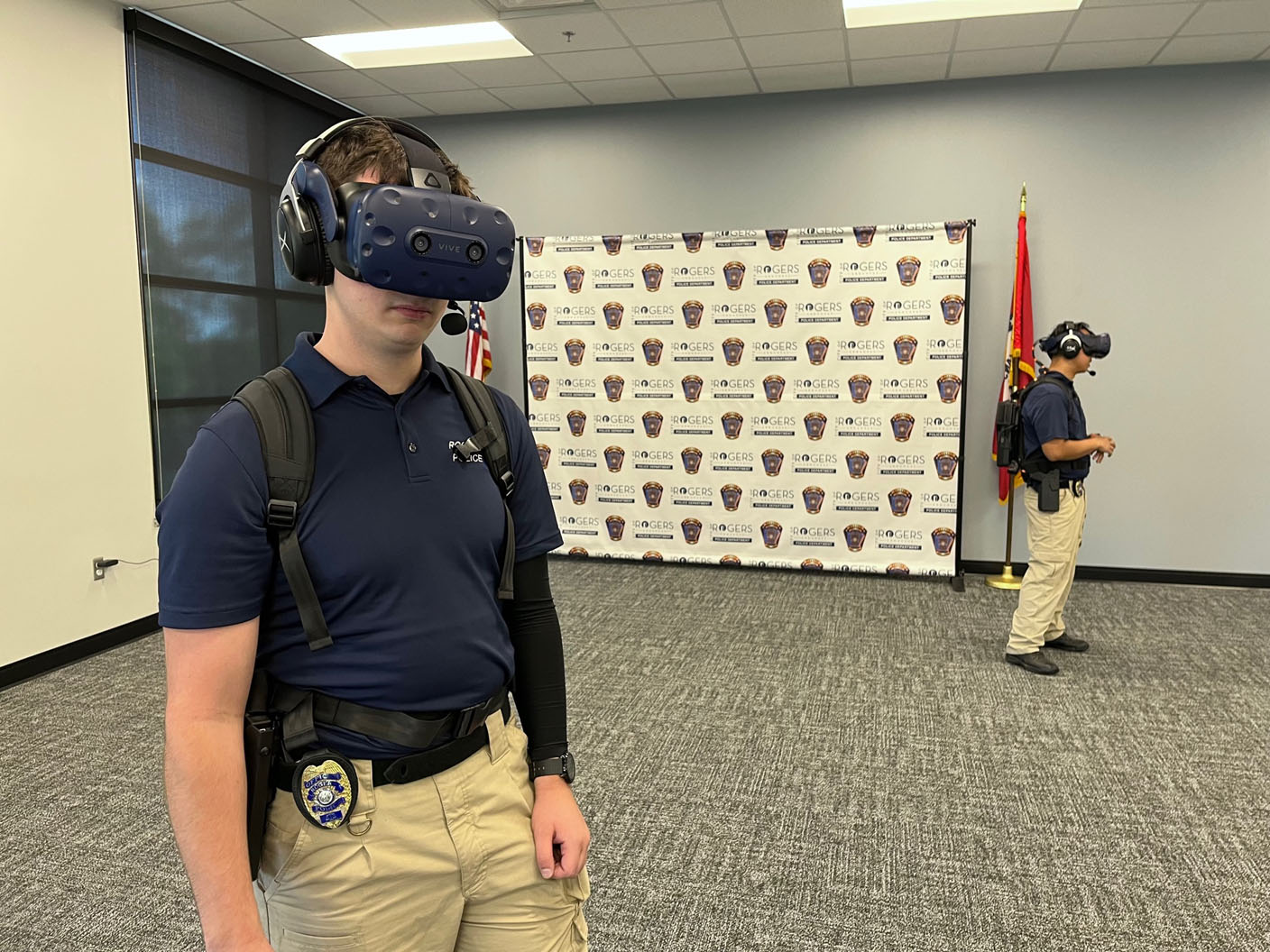The photograph depicts two young men, possibly teens or young adults, standing in a room with an office-like ambiance. Both are dressed in matching uniforms consisting of blue, short-sleeved, collared shirts and khaki pants. Each wears a police badge on their right hip and a black belt, though only the individual on the left has a visible badge. They are accessorized with black shoes and black backpacks with visible straps. Both are utilizing advanced virtual reality headsets, identified as HTC Vive models, equipped with headphones and microphones positioned over their mouths.

The room features a drop ceiling with the typical office tile pattern and fluorescent lighting. The floors are carpeted in a gray and white pattern, and the walls reflect a mix of gray and tan hues. To the back left, a window is covered by a blackout shade, and next to it is a backdrop designated for photo shoots, emblazoned with repeated police badges and the name "Rogers." The backdrop is flanked by two flags: an American flag partially visible on the left, and another red flag to the right, both supported by brown rods with brass bases.

Closely examining the VR setup, the individual on the left, partially obscured, shows additional details like a black sleeve covering his left arm, while the individual on the right has more visible components such as his black shoes and a holstered gun. Both men maintain a neutral expression as they engage with the virtual reality environment.